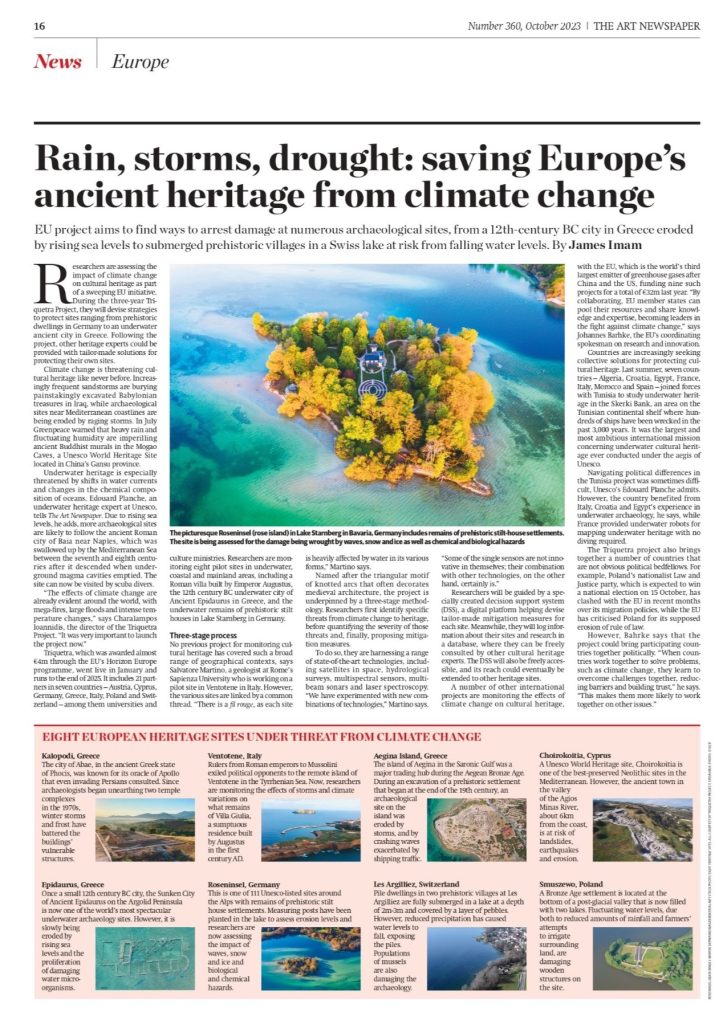Caption: A detailed screenshot of a web page formatted like a traditional newspaper. The page is from "The Art Newspaper," dated October 2023, specifically from page 16, issue number 360, under the section "News Europe." Dominating the page is the headline article titled "Rain, Storm, Strout: Saving Europe's Ancient Heritage from Climate Change" by James Imam.  The piece delves into an EU project focused on mitigating climate damage to various archaeological sites, ranging from a 12th century BC city in Greece threatened by rising sea levels to submerged prehistoric villages in Switzerland endangered by falling water levels. The centerpiece of the article is a vivid image of a small island surrounded by clear turquoise water, with its foliage displaying autumnal shades of yellow and green. Framing the article are columns of text that remain too small to decipher. Below, another article titled "8 EU European Heritage Sites Under Threat from Climate Change," showcases images and descriptions of eight threatened heritage sites, all visually linked to water, although the details remain indistinct due to the small text size. The overall background of the page is white, enhancing the traditional newspaper aesthetic.